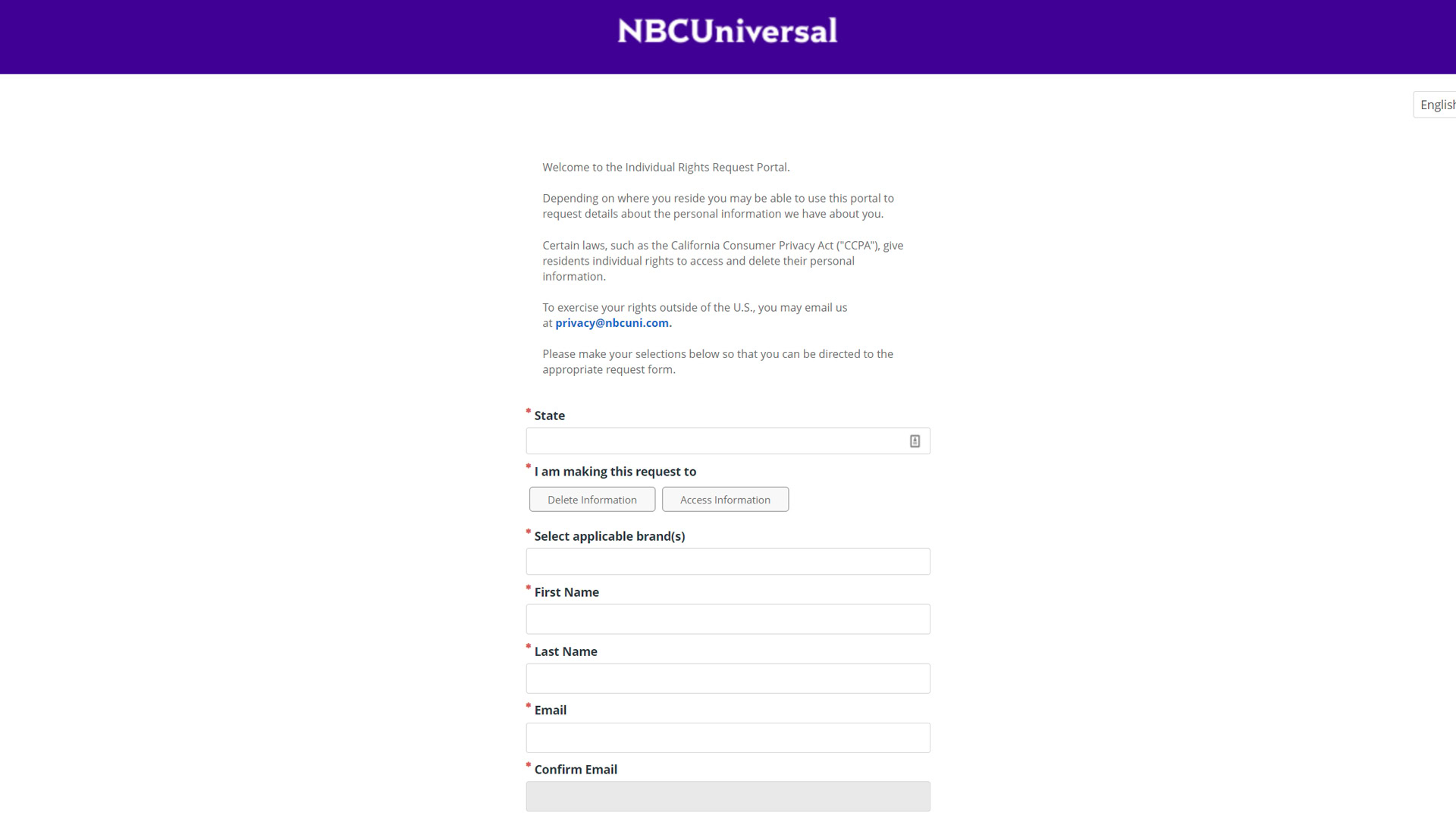The image displays a prominent blue box at the top of the screen with "NBC Universal" written in bold letters. Below this, the background shifts to an all-white color. The text on this white background reads, "Welcome to the Individual Rights Request Portal." The message explains that, depending on your place of residence, this portal can be used to request details regarding your personal information. It mentions that certain laws, such as the California Consumer Privacy Act (CCPA), grant residents specific rights to access and delete their personal data.

For users outside the U.S., it instructs them to email privacy@NBCUNI.com to exercise their rights. The portal prompts users to make selections to be directed to the appropriate request form. The first prompt asks users to select their state of residence and whether they are making a request to either delete or access information. The form then asks for applicable brands, followed by fields for the user's first name, last name, and email address, ending with a gray box to confirm the email. Notably, required fields have a red asterisk next to them.